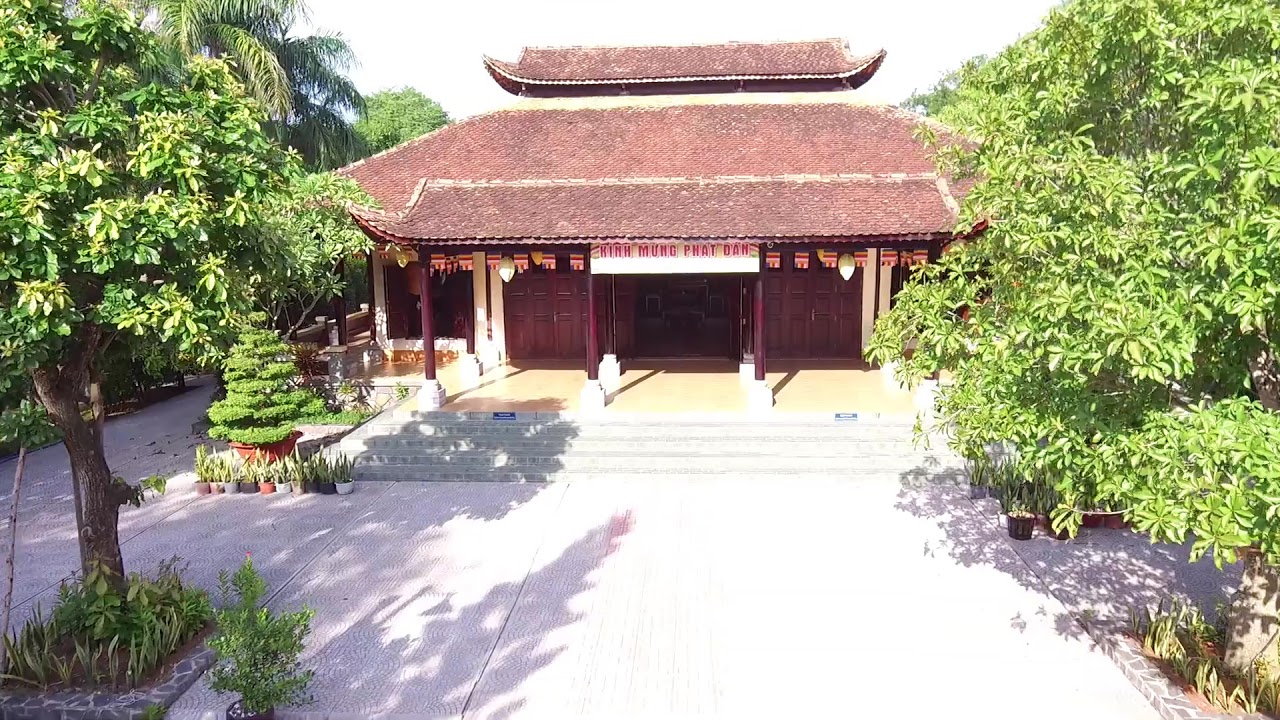This image depicts an intricately designed Asian temple, reminiscent of a pagoda, set against a bright, sunny sky that almost appears white due to the intense sunlight. The structure primarily showcases the lower floor and a glimpse of the next level's curved roof, characterized by its upward-arching corners and covered in reddish tiles. The front of the building is adorned with red panels and white beams, with concrete pillars supporting the entrance. 

Leading up to the temple, a few steps and a small landing area are paved with neatly arranged cement squares, creating a gleaming white courtyard due to the strong sunlight. To either side of the temple, there are well-maintained deciduous and tropical trees, some potted and finely trimmed to maintain a tidy appearance, adding a touch of nature to the scene. 

The front facade of the temple features a white sign with red writing, possibly spelling out "KIMH MUNG PHAT DAN." Additionally, banners and lanterns drape across the entrance, enhancing the cultural ambiance. Shadow play from the sunlight indicates clear skies, casting distinct shadows around the area.